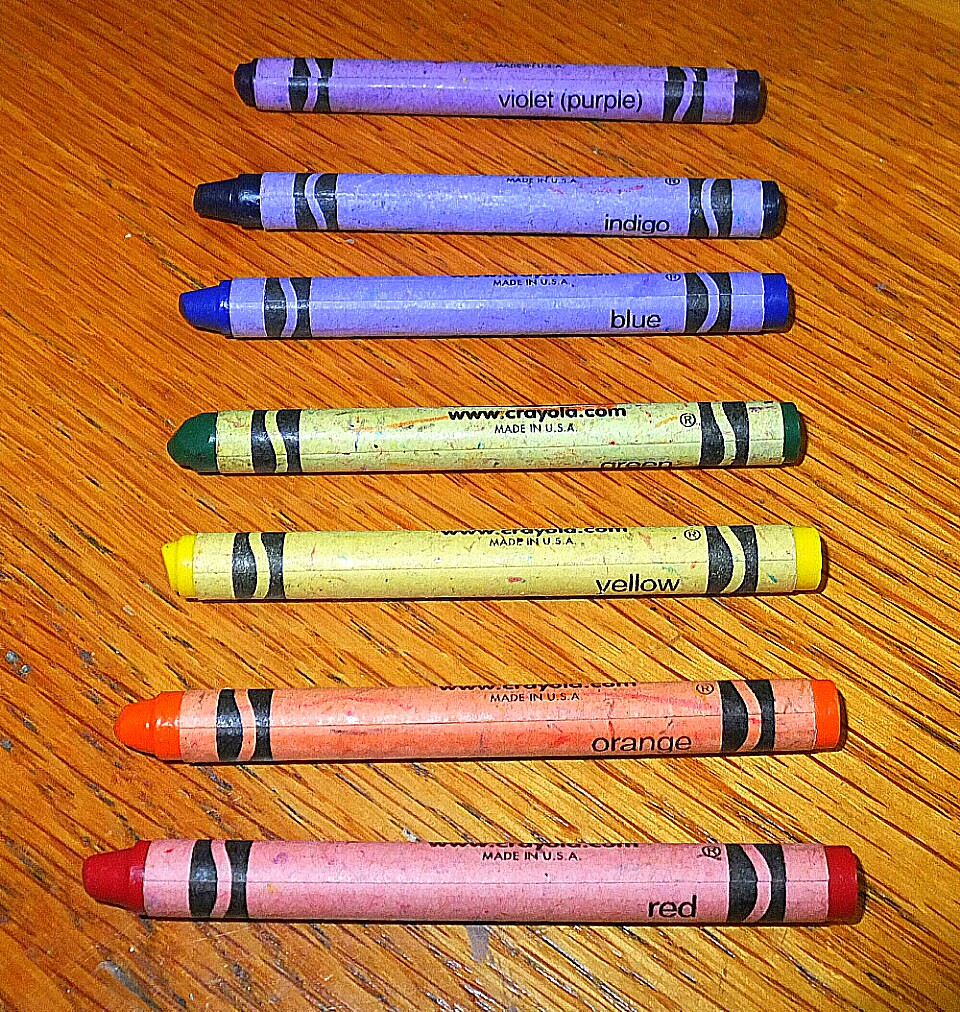This close-up photograph features seven Crayola crayons neatly lined up on a light brown wooden table, captured with such detail that the wood grain is visible. The bright flash used in a darker setting gives a stark brilliance to the image. The arrangement of the crayons flows from the top of the photograph to the bottom, starting with violet (purple) on the top, followed by indigo, blue, green, yellow, orange, and ending with red closest to the viewer. Each crayon shows signs of use: the violet crayon is barely worn, while the green and yellow crayons have their tips significantly worn down. The orange and red crayons appear moderately used. On the crayon wrappers, traces of other colors indicate they were likely stored together in a container. The image is well-framed, highlighting the everyday beauty of these well-loved art supplies.